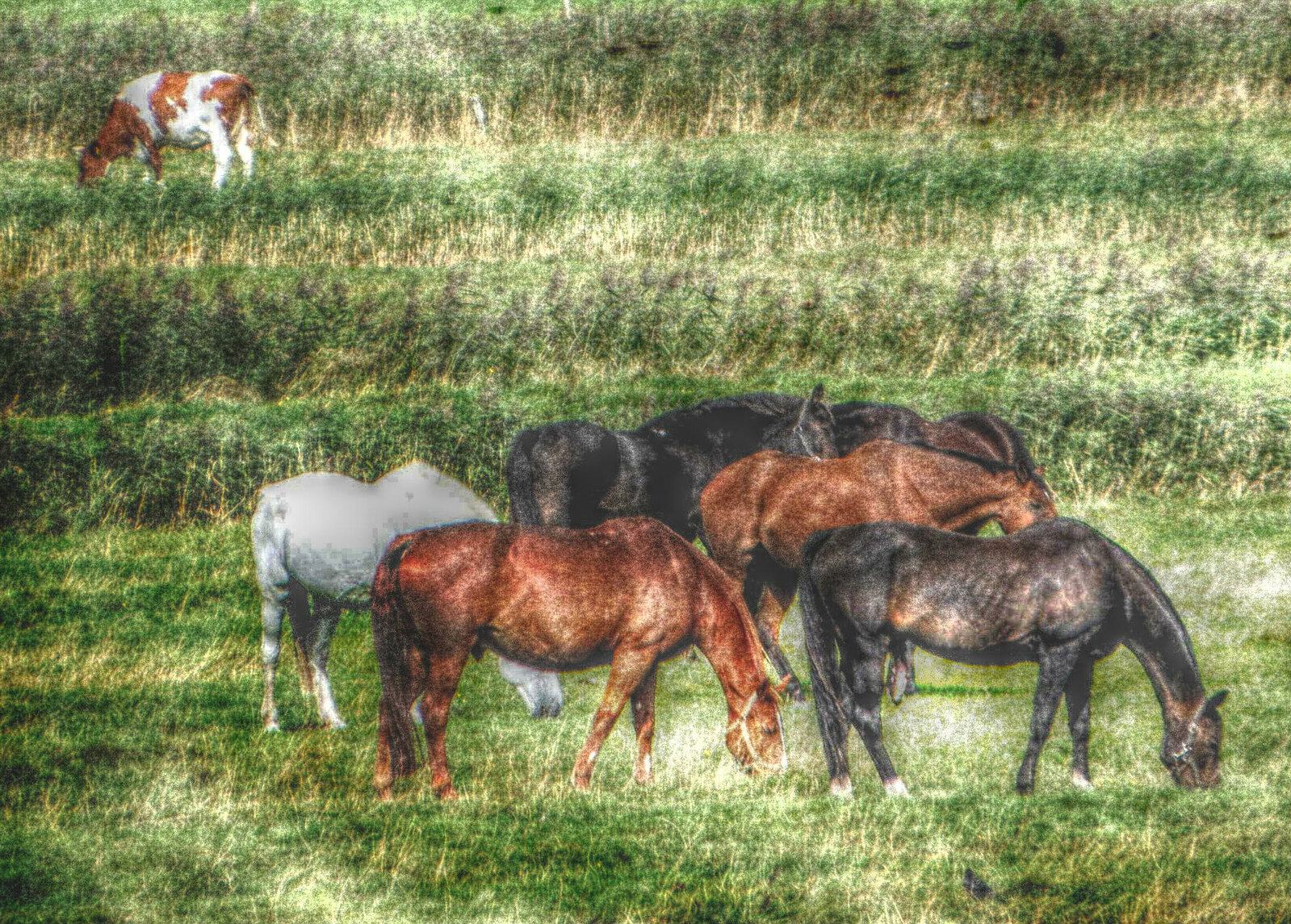The image is a detailed and vibrant painting, possibly on a textured medium like velvet or a throw blanket. It depicts a serene pastoral scene with a small herd of six horses and a cow in a green pasture. The horses, positioned in the foreground, are grazing with their heads down. They consist of three black horses, two brown horses, and one white horse. The brown and black horses have some variations in their shades, with some showing lighter patches or splotches around the midsections. The cow, located in the upper left-hand corner of the image, has a distinctive white coat with brown spots and is also grazing. The pasture itself is lush with predominantly green grass interspersed with patches of yellowish, dried grass, giving a realistic textural depth. The background features slight rolling hills and rows of green crops or ridges, enhancing the bucolic setting. The sunlight casts varied shading, producing bright and shadowy areas that add to the painting's depth and dynamism.